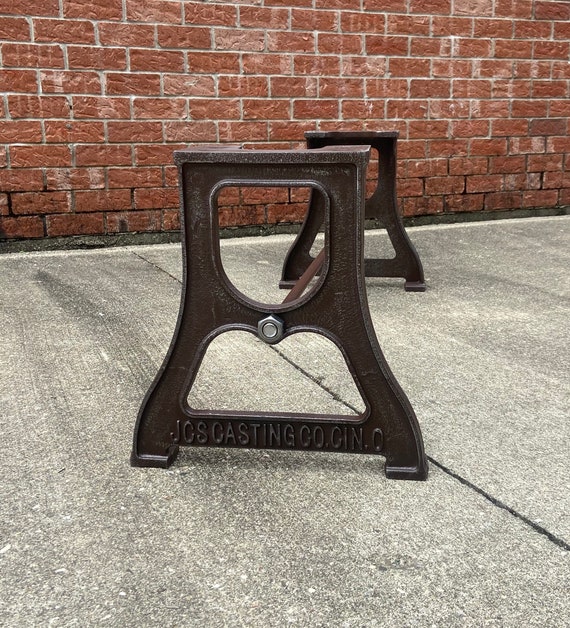The image depicts a cast iron-style bench frame, likely intended to form the legs and support structure of a park bench. The bench lacks the wooden planks that would typically form the seat and backrest. The cast iron is brown in color and features an engraving on the side that reads "JCS Casting Company CIN." The design is flat at the top and widens towards the base of the feet. A silver bolt and nut connect a brown metal rod to another identical part of the frame, suggesting that these components are the support legs of the bench. The frame rests on a gray concrete floor, while a red brick wall serves as the backdrop.